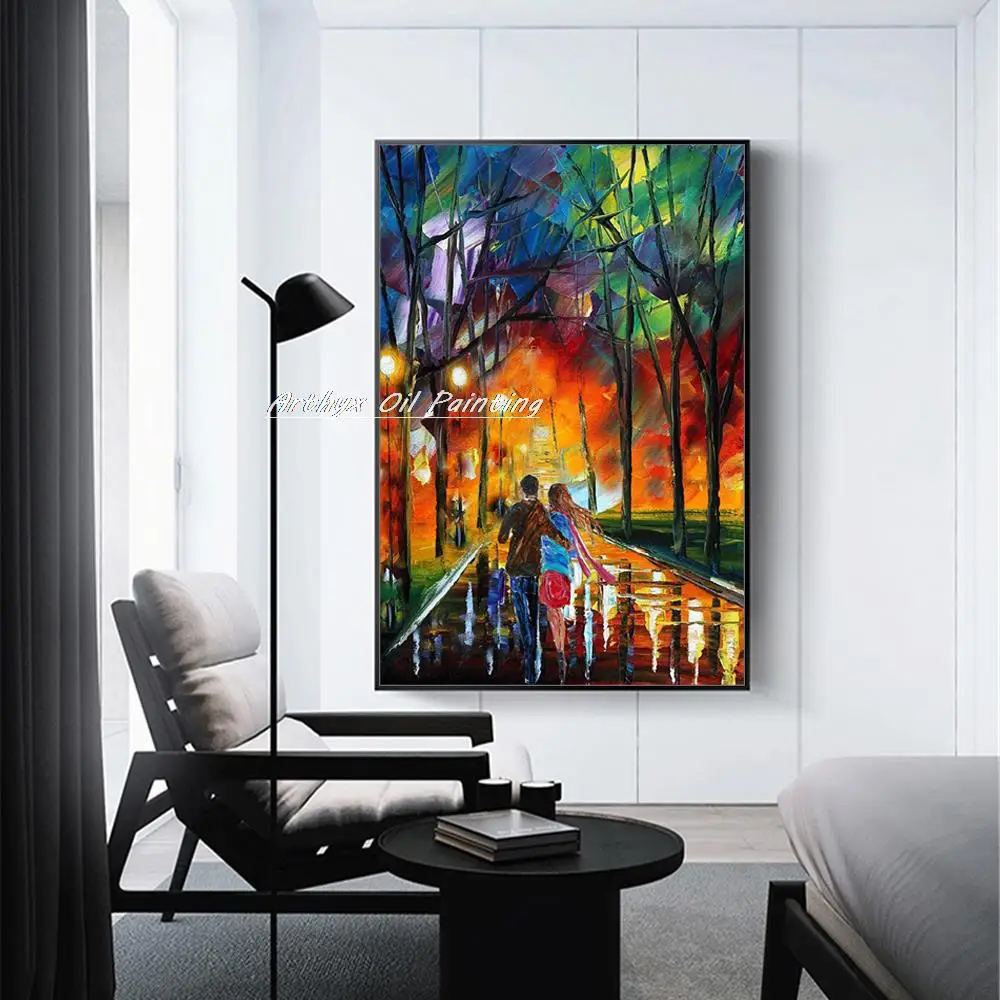This image depicts a modern, indoor room featuring a colorful and vibrant oil painting on a white paneled wall. The painting, framed in black and watermarked with "ARTHYX OIL PAINTINGS," portrays a man in a brown jacket with his arm around a woman in a blue shirt and red skirt, as they walk down a warm-hued street shaded by trees with leaves in an array of colors including green, purple, orange, red, and yellow. The room itself has white walls with a large window on the left, draped with a black curtain that allows sunlight to stream in. Furnishings include a black Adirondack chair with a white cushion, a black circular table that holds two books, a black floor lamp, and a black-framed bed with white sheets positioned in the corner. The scene is further completed with a gray rug underfoot and other pieces of furniture subtly visible, reinforcing the room's contemporary aesthetic.